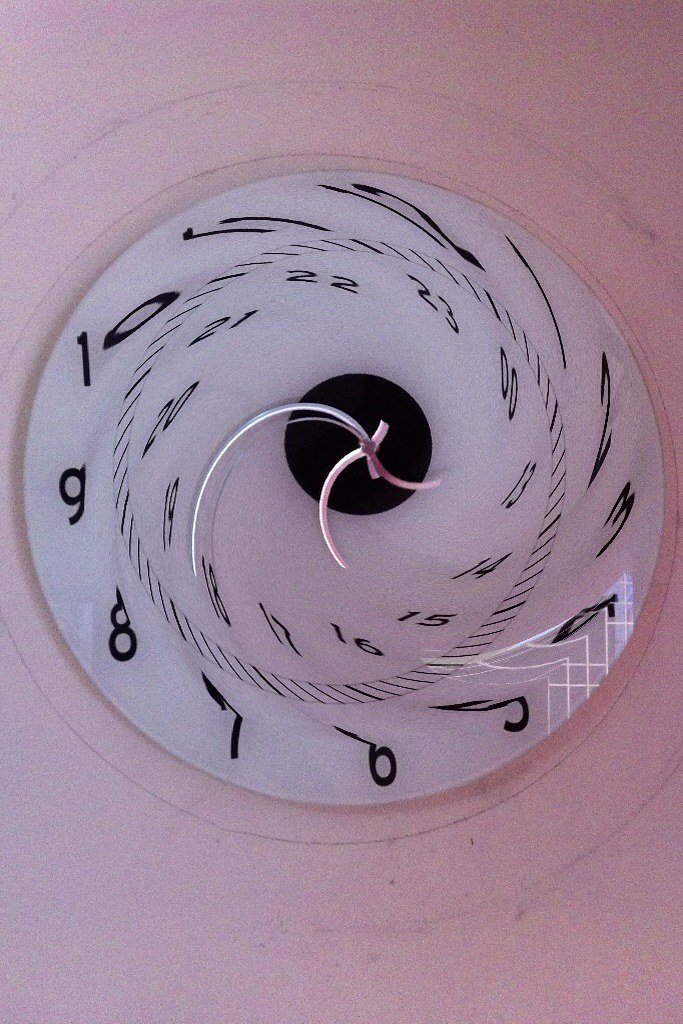The image features a modern and visually striking clock mounted on a wall with a pink, blotchy background adorned with pencil-drawn circles. The clock itself has a white face and a black central circle where the clock hands are attached. The black digits appear distorted and stretched, almost as if they are caught in a vortex or whirlpool. Numbers 1 through 6 seem to spiral outward, becoming more distorted as they progress clockwise, while numbers 7, 8, 9, and 10 are slightly less stretched but still noticeably altered. Inside the clock face, additional numbers ranging from 0 to 23 are also present and follow a similar distorted pattern. The clock hands, which are silver and white, are curved and warped to match the swirling aesthetic of the digits, adding to the overall sense of the clock being caught in a dynamic, almost chaotic motion.